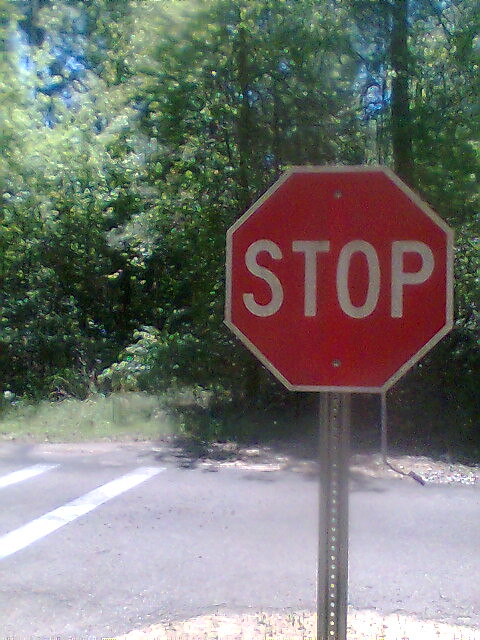This vibrant color photograph captures a daytime outdoor scene at a T-intersection, viewed from directly in front of a stop sign. The road ahead ends in a dead-end, with directions only allowing for a left or right turn. Across the street, a lush expanse of green trees dominates the view, hinting at a serene, natural environment. A possible trail seems to weave through the trees on the left side, adding an element of exploration to the scene. A crosswalk is visible on the left, indicating pedestrian pathways and access. At the very bottom of the image, the stop sign's pole extends down to a curved dirt patch, marking the corner of the intersection.